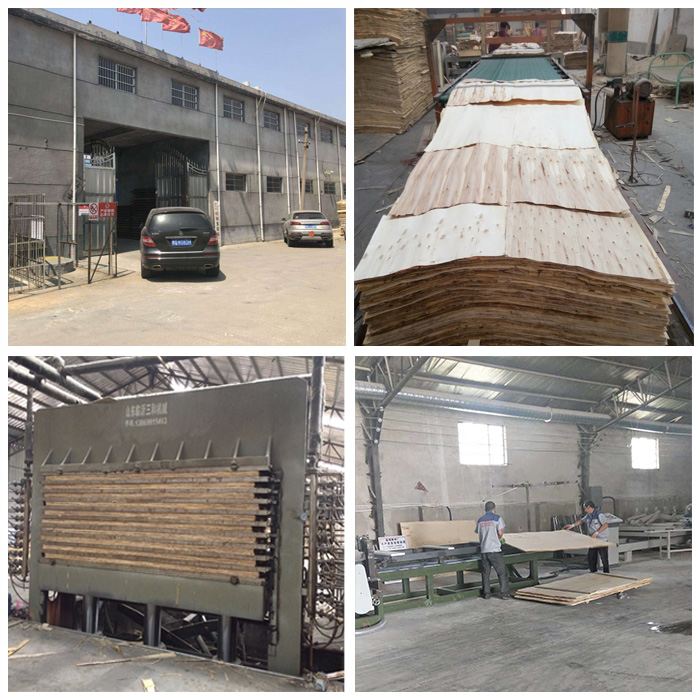This image is a collage consisting of four separate yet related photos, arranged in a windowpane format. In the upper left quadrant, a couple of cars are parked outside a gray, two-story warehouse or factory building, distinguished by several red Chinese flags above the entrance and barred windows. The upper right quadrant appears to show the inside of this building, with stacks of wood or some form of building materials or textiles neatly organized. The lower left quadrant contains a large, somewhat indistinct metallic machine, potentially part of the production process, with scraps of wood or fabric scattered below it. In the lower right quadrant, factory workers dressed in gray pants and alternating light blue and dark blue shirts with red writing are busy handling a large piece of wood on a table, either placing it on or removing it from a stack. The overall setting and elements suggest that this facility is involved in woodworking or wood processing. The color palette includes shades of blue, red, tan, brown, black, silver, and green.